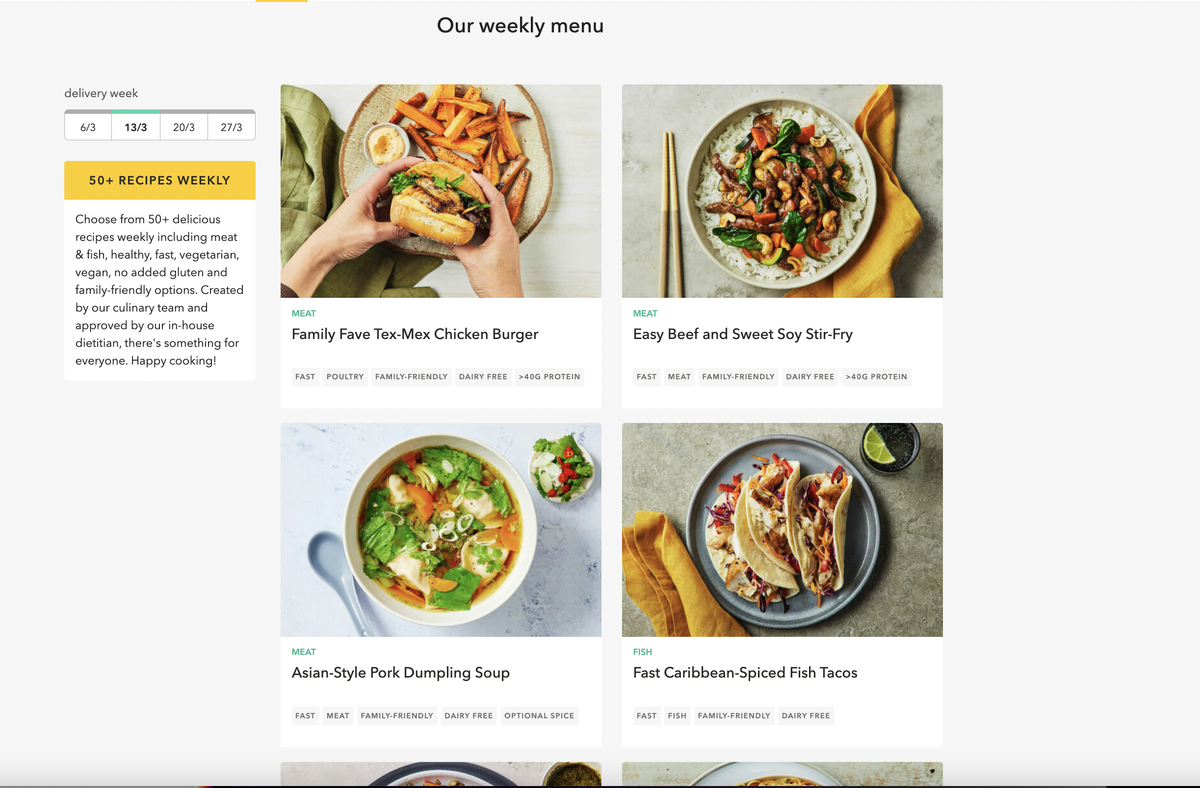This promotional image from a meal delivery service features an off-white background. At the top, the text "Our Weekly Menu" is prominently displayed. On the upper left side, a section titled "Delivery Week" offers four options: 6-3, 13-3, 20-3, and 27-3, with the date 13-3 highlighted by a green bar above it.

Beneath this section, a white rectangular box with an orange banner at the top contains the text: "50-plus recipes weekly. Choose from 50-plus delicious recipes weekly, including meat and fish, healthy, fast, vegetarian, vegan, no added gluten, and family-friendly options. Created by our culinary team and approved by our in-house dietitian. There's something for everyone. Happy cooking."

The main portion of the image showcases four recipe options accompanied by their representative images. These include "Family Fave Tex-Mex Chicken Burger," "Easy Beef and Sweet Soy Stir-Fry," and "Asian-Style Pork Dumpling Soup" in the meat category, as well as "Fast Caribbean Spiced Fish Tacos" in the fish category.